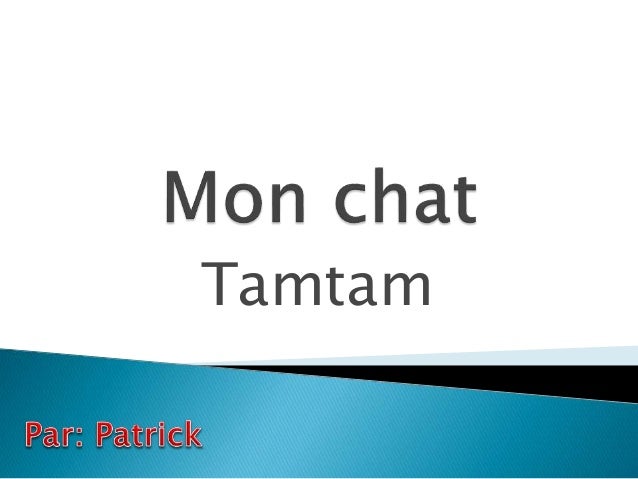The image features a central title that reads "Monchat Tam Tam" in dark grey letters against a clean white background. Beneath this title, a prominent blue slope stretches from the left to the right of the image, forming an irregular quadrilateral with a diagonal top edge. Adorning the middle part of this blue slope near the left are two smaller triangles—one light blue and the other black—protruding to the right. Situated in the lower left corner of the blue slope, a red inscription reads “Par : Patrick” with white outlines. The composition is visually dynamic with the use of contrasting colors and geometric shapes, evoking an impression of modern digital graphics.